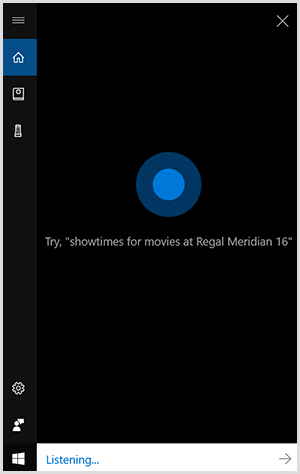This is a detailed screenshot of a smartphone interface, likely captured during a voice-activated search. The screen's background is entirely black. In the upper left-hand corner, a gray hamburger menu icon is displayed, which users can click for additional options. Directly across from it, on the right side, is a gray 'X' icon. 

Beneath the hamburger menu, aligned to the left, is a highlighted 'Home' button encased in a blue box, indicating that the home screen is currently active. Below this, there are two additional icons, though their functions are not immediately identifiable. Continuing down the left side, a black bar runs the full length, featuring several more icons: a settings icon, an avatar icon with an adjacent element, and the Microsoft logo in white.

In the center of the screen, there is a visual composed of a medium blue circle encircled by a dark slate blue ring. Below this image, gray text reads: "try 'show times for movies at Regal Meridian 16.'" This suggests that the user may have issued this voice command. At the bottom, a blue bar displays the word "Listening," indicating that the device is currently processing a voice query.